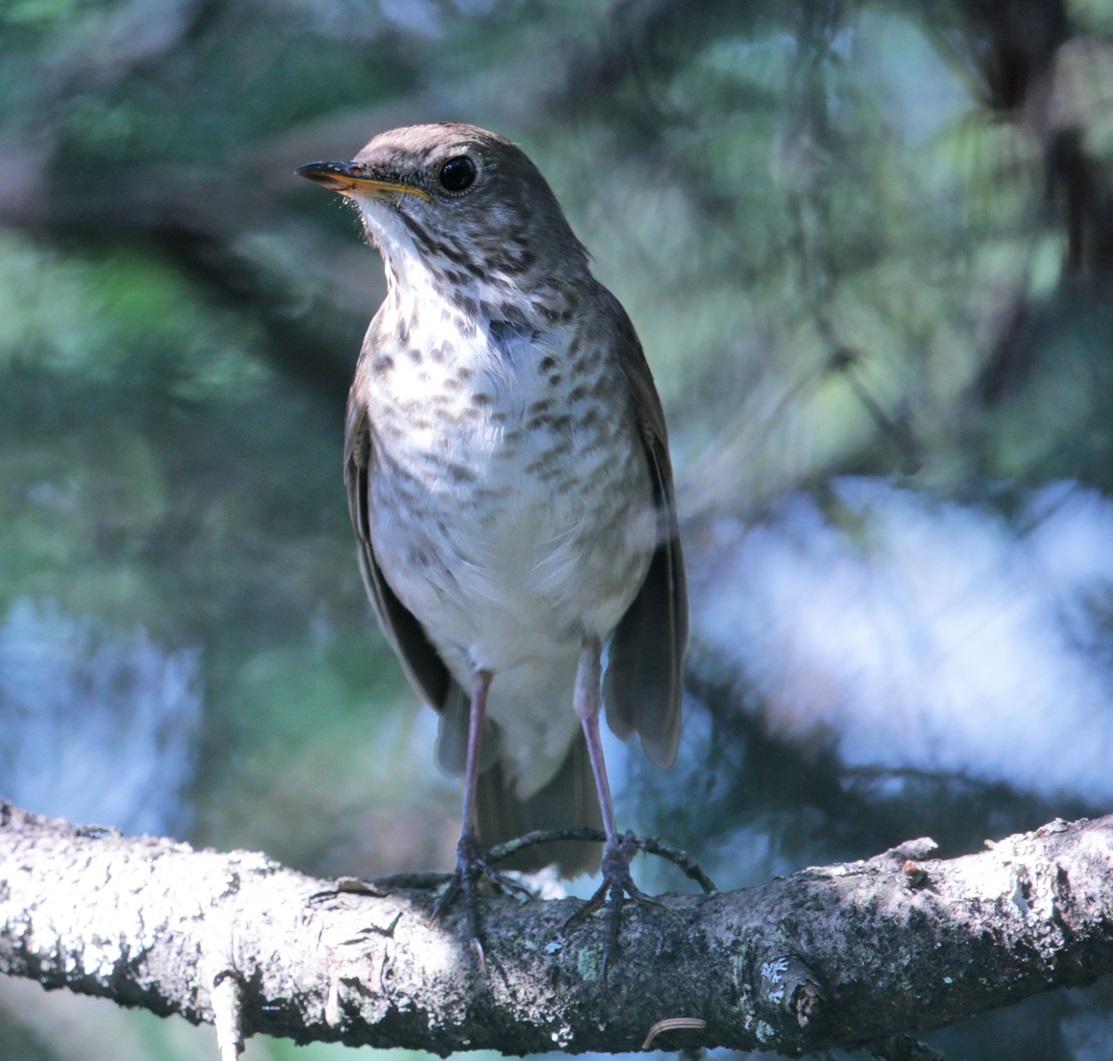This image, likely a lifelike painting or a high-quality photograph, depicts a young bird standing on a slightly curved branch, positioned centrally against a blurry outdoor background. The background, out of focus with a bokeh effect, reveals hints of green foliage, blue sky, and possibly pine needles. The bird, which appears to be set in the middle of the day, displays a mix of colors: its head and body are adorned with brown and grayish-brown speckles, it has a white belly, and its wings are folded behind its back. The bird features big black eyes, a black beak with yellow accents, and legs that appear white near the body but transition to dark gray down to the feet. The bark of the branch similarly exhibits varying shades from light due to illumination to darker grays. The intricate details of the bird, combined with the natural surroundings hinted at in the blurred background, create a detailed and captivating portrayal of nature.